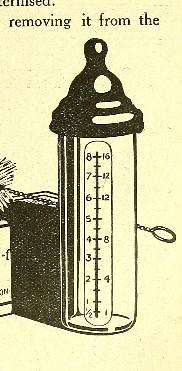A cropped, sepia-toned image extracted from an old book, showcasing an empty baby bottle adorned with a rubber nipple. The baby bottle displays measurement markings along its side. Behind it, a wire cleaning brush can be partially seen. The composition includes fragments of a plain box and another box with indistinguishable text, but the focal point remains on the baby bottle and its immediate surroundings. The surrounding text from the original source has been truncated, contributing little context to the image other than recognizing the depicted baby bottle and cleaning brush.